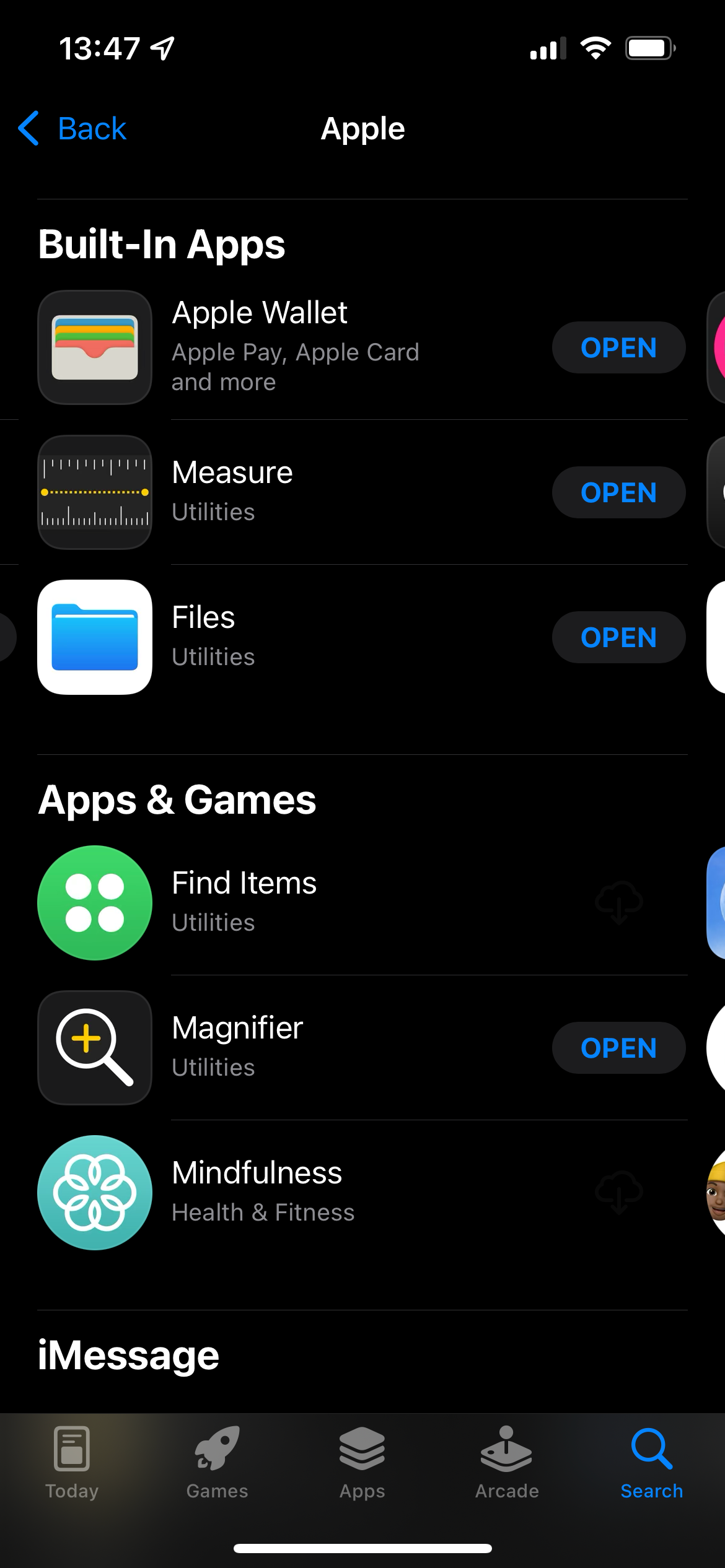This is a screenshot from a smartphone screen, featuring predominantly black, white, and blue text, as well as various icons and logos. At the top, the time is displayed as 13:47, with accompanying Wi-Fi and battery icons situated to the right. Beneath the time, there is a left-facing arrow icon labeled "Back" in blue.

In the main content area, there is a white Apple logo followed by the text "Built-in Apps." The first listed app is "Apple Wallet," with a corresponding Apple Wallet logo. Under this category, features such as Apple Pay and Apple Card are mentioned. To the right of this entry, there is a partially visible "Open" button.

The next app listed is "Measure" within the Utilities category, accompanied by its respective logo and an "Open" button that is also partially cut off.

Further down, the "Files" app is listed under Utilities, with its logo and a full "Open" button visible to the right.

Below that, under the Apps and Games section, the "Find Items" app is displayed with its Utilities tag and logo, though the "Open" button is cut off at the right edge of the screen.

Next, the "Magnifier" app is listed under Utilities with an associated icon and a visible "Open" button.

Following that is the "Mindfulness" app under the Health and Fitness category, with its logo. There is no "Open" button visible next to this entry, as it is cut off.

At the bottom of the screen, the iMessages app is noted, and the navigation tabs for Today, Games, Apps, Arcade, and Search are displayed, with the Search tab currently active.